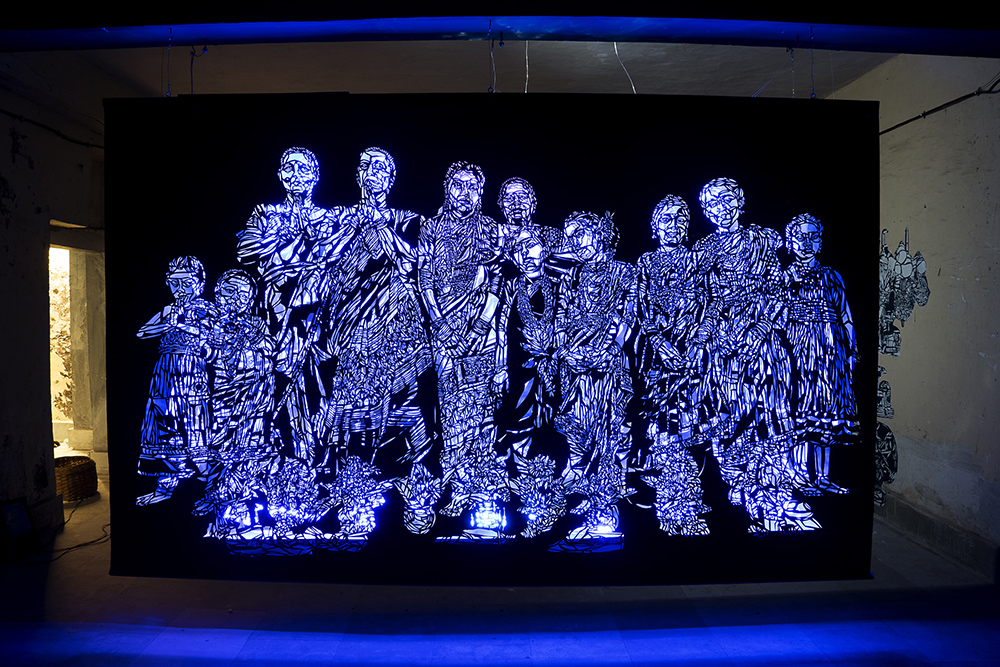In this image, we observe a captivating art installation that utilizes illuminated lights, giving it an ethereal glow that suggests it may not exist in the same way without the lighting. The artwork is displayed against a stark black background, accentuating the luminous figures that populate the scene. Among these figures, we see depictions of humans, both children and adults, arranged at various positions within the frame. Some of the figures appear fragmented, as if made from shredded paper, while others are fully intact. Despite their fragmented or whole forms, all the figures feature carefully designed faces. The characters seem to belong to an ancient tribe, adorned with robes and cloth wraps around their shoulders and waists. They are depicted in various gestures, some appearing to pray. The predominant hues of blue and white, enhanced by the blue lighting in the room, create a holographic effect, making the figures appear multidimensional and almost lifelike. This holographic illusion, combined with the positioning of about ten characters facing the viewer, contributes to the overall mesmerizing and intricate nature of the installation.